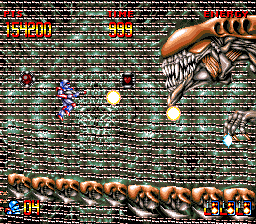This detailed image captures the nostalgic essence of an old-school computer game from the 80s or 90s, likely played on an original NES system. It freeze-frames an intense action sequence: a main character, depicted as a blue-suited figure, is mid-air, either jumping or floating, while firing a weapon that emits two round balls of light. This character is situated in the middle-left of the image. The target of his attack is a formidable alien boss, entering from the right side of the screen. The alien boasts a bronze carapace, jagged teeth, and a segmented, armor-like tail wrapping around the bottom of the screen. A bony hand from the alien also appears, adding to its menacing presence. The backdrop features a checkered pattern with black and green squares, and the interface is rich with game information: the upper left corner displays a score of 154200 in striking red and yellow digits, and the time is marked as 999. Additionally, the lower left shows '04' beside an avatar of the player, indicating four lives remaining. Energy status is noted but appears to be dangerously low, as no energy bars are visible.